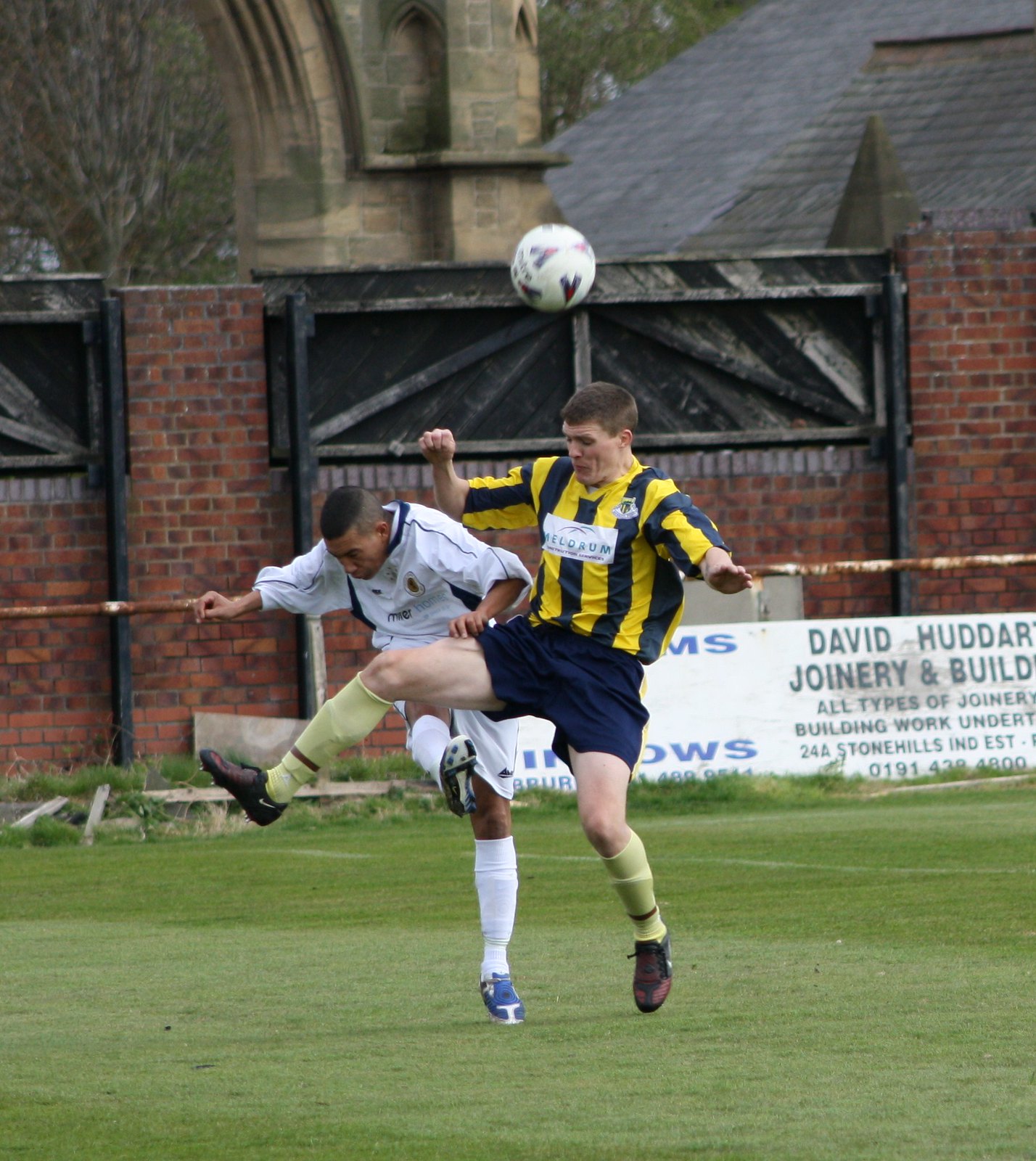The image captures an intense moment between two soccer players vying for possession of the ball, which is aloft above their heads. The player in the foreground is wearing dark blue shorts, light green socks, and brown shoes. His shirt is yellow with dark blue stripes. He appears to have just headed the ball. The player behind him, dressed predominantly in white with subtle blue accents, including a dark blue collar, has his right leg kicked upwards. They are both playing on well-maintained grass. The setting includes a brick building and an archway in the background, accompanied by a sign that partially reads "David Hadar joinery and building," suggesting a construction company sponsorship. The action likely takes place in the middle of the day, as evidenced by the good lighting conditions.